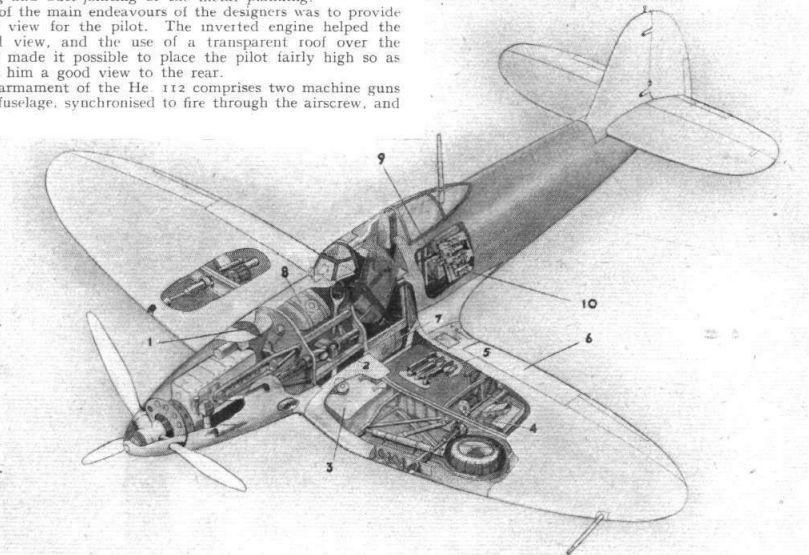This image features a vintage, hand-drawn, pen-and-ink sketch of a World War II Spitfire aircraft, depicted at a diagonal angle, allowing visibility of nearly all aspects of the plane. The illustration is highly detailed, showing a cross-sectional view that exposes both internal and external parts, including the propellers, interior wing structures, and the canopy. The drawing is annotated with numbers and lines pointing to various components, facilitating a thorough understanding of the aircraft's design.

A snippet of contextual text is visible in the upper left corner, albeit partially obscured. It reads: "of the main endeavors of the designers was to provide view for the pilot. The inverted engine helped the view and the use of a transparent roof made it possible to place the pilot fairly high so as to give him a good view to the rear." The monochrome palette of the image, featuring shades of black, white, and gray, suggests the illustration is a photocopy possibly taken from an old textbook or diagram. 

Overall, the central position of the aircraft and the meticulous detailing emphasize the technical and historical significance of the design elements highlighted in the diagram.